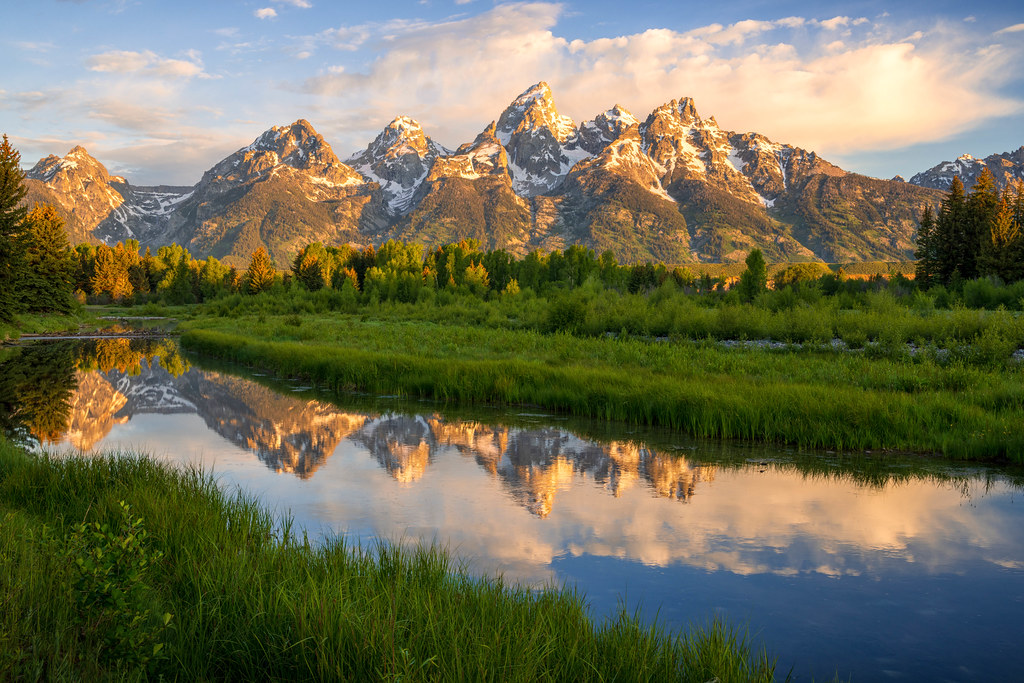The image captures a breathtaking mountainscape, either a photograph or a meticulously detailed painting, viewed from a valley below. The backdrop features towering mountains with snow-capped peaks beneath a vivid, almost piercingly blue sky adorned with scattered, white, puffy clouds. The weather looks perfect, with the sky appearing lighter on the right side, hinting at the sun partially obscured by a cloud.

In the foreground, a serene body of water—possibly a stream or small lake—perfectly mirrors the majestic mountains and the clouds above, enhancing the image's striking beauty. The water's surface is smooth and crystal clear, offering an undisturbed reflection.

Between this tranquil water and the imposing mountains lies a lush expanse of greenery: tall grass, verdant trees, and bright green grass especially vibrant in the bottom left of the image. This rich tapestry of natural elements contributes to the scene’s overall picturesque and tranquil atmosphere.